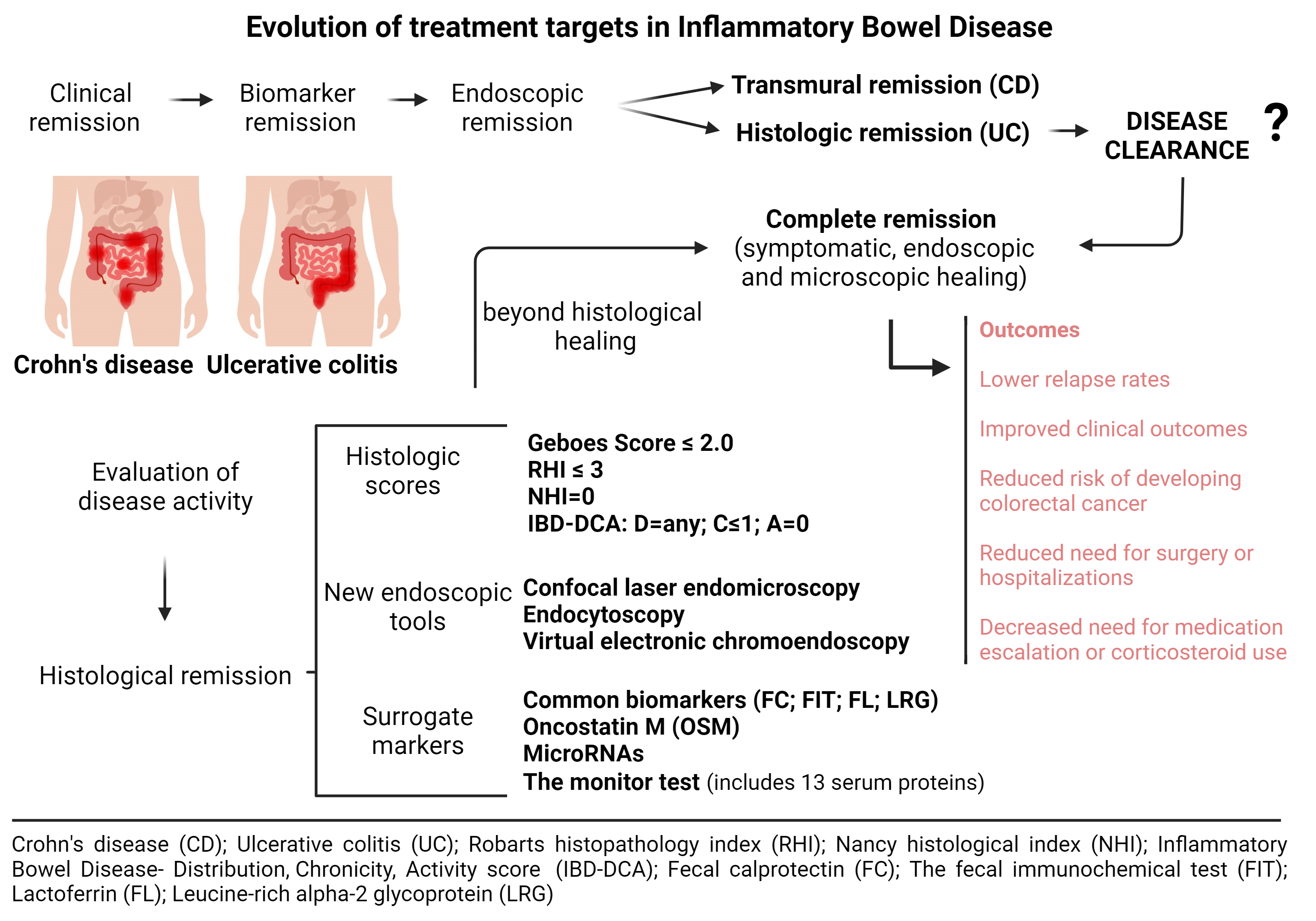The image is a detailed medical poster displayed in a physician's office, titled "Evolution of Treatment Targets in Inflammatory Bowel Disease" in black bold letters at the top. This oblong poster features a flowchart that visually outlines the stages and targets of treatment for inflammatory bowel diseases, specifically Crohn's disease and ulcerative colitis.

At the very top, the flowchart starts with "clinical remission," leading sequentially through "biomarker remission" and "endoscopic remission." It further branches into "transmural remission (CD)" and "histologic remission," ultimately culminating in "disease clearance" and "complete remission" with a question mark. Complete remission encompasses "symptomatic, endoscopic, and microscopic healing."

Central to the poster, two cutaway illustrations of the human abdomen depict the affected areas of Crohn's disease on the left and ulcerative colitis on the right, highlighted in pink and red. These images are accompanied by information on evaluating disease activity and detail various remission targets such as histological scores, new endoscopic tools, and surrogate markers, leading towards "beyond histological healing."

The bottom section of the poster describes the positive outcomes associated with achieving these treatment targets, including lower relapse rates, improved clinical outcomes, reduced risk of developing colorectal cancer, decreased need for surgeries or hospitalizations, and a reduced need for medication escalation or corticosteroid use, all indicated in pink.

In summary, the poster provides a comprehensive and sequential guide to the treatment targets and outcomes for Crohn's disease and ulcerative colitis, emphasizing the pathway from initial clinical remission to complete remission and the benefits of achieving these targets.